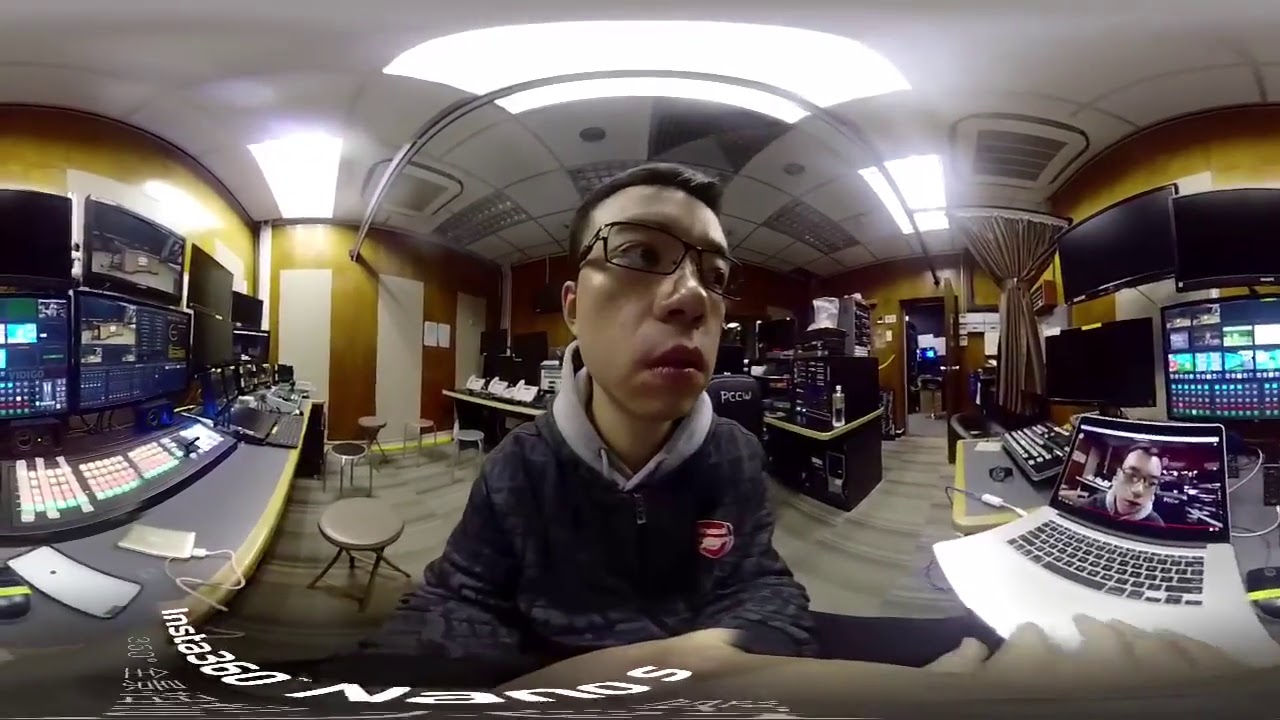The image is a horizontally-oriented, convex photograph capturing a man in what appears to be a technology-driven environment, possibly a recording studio or control room. The unusual lens distorts the scene into circular shapes, giving it a unique appearance. At the center, the man is seated on a stool, identifiable by his glasses and brown rain jacket. His expression is somewhat serious. In front of him, there's unreadable writing and his image is also displayed on a laptop screen situated to the right, adding a layer of digital interaction to the scene. The room is filled with various electronic equipment and computer systems, with a notable keyboard-like device to the left that might be used for music manipulation. The setting includes multiple gray stools scattered around a similarly gray floor, a portion curtained off with held-together drapes, and numerous display monitors on the walls. Overhead, the ceiling is white with fluorescent lighting, illuminating the technologically rich ambiance.